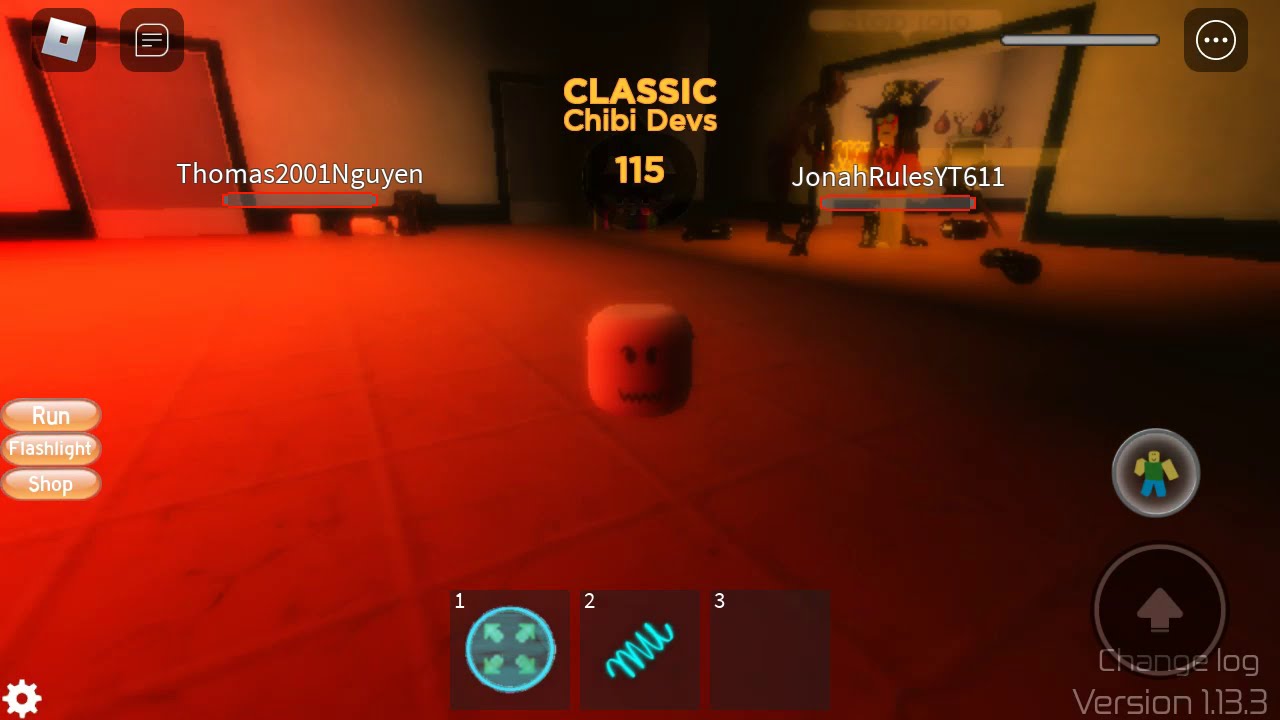In this screenshot from a video game, we see a detailed room illuminated by a vibrant red light originating from the top left-hand corner, casting a glow onto a tiled stone floor. The room has walls to the left and right, with the right wall featuring a large opening that leads to another area. In the foreground on the floor, a marshmallow-shaped character with a face—two eyes and a mouth—faces the camera. Above it, yellow text reading "Classic Chibi Devs 115" is arranged in three lines. 

The interface is bustling with elements: a small inventory pane with three transparent squares is visible at the bottom, with two of them containing symbols. The lower left corner shows a white gear icon, while higher up on the left are three oval buttons labeled "run," "flashlight," and "shop." On the lower right, a circular icon with an arrow and a smaller circle with a human figure can be seen. Additionally, username-style texts appear in white, with "Thomas2001Nguyen" and "JonahRulesYT611" among them. The atmosphere suggests a colorful and animated style, likely appealing to a younger audience.